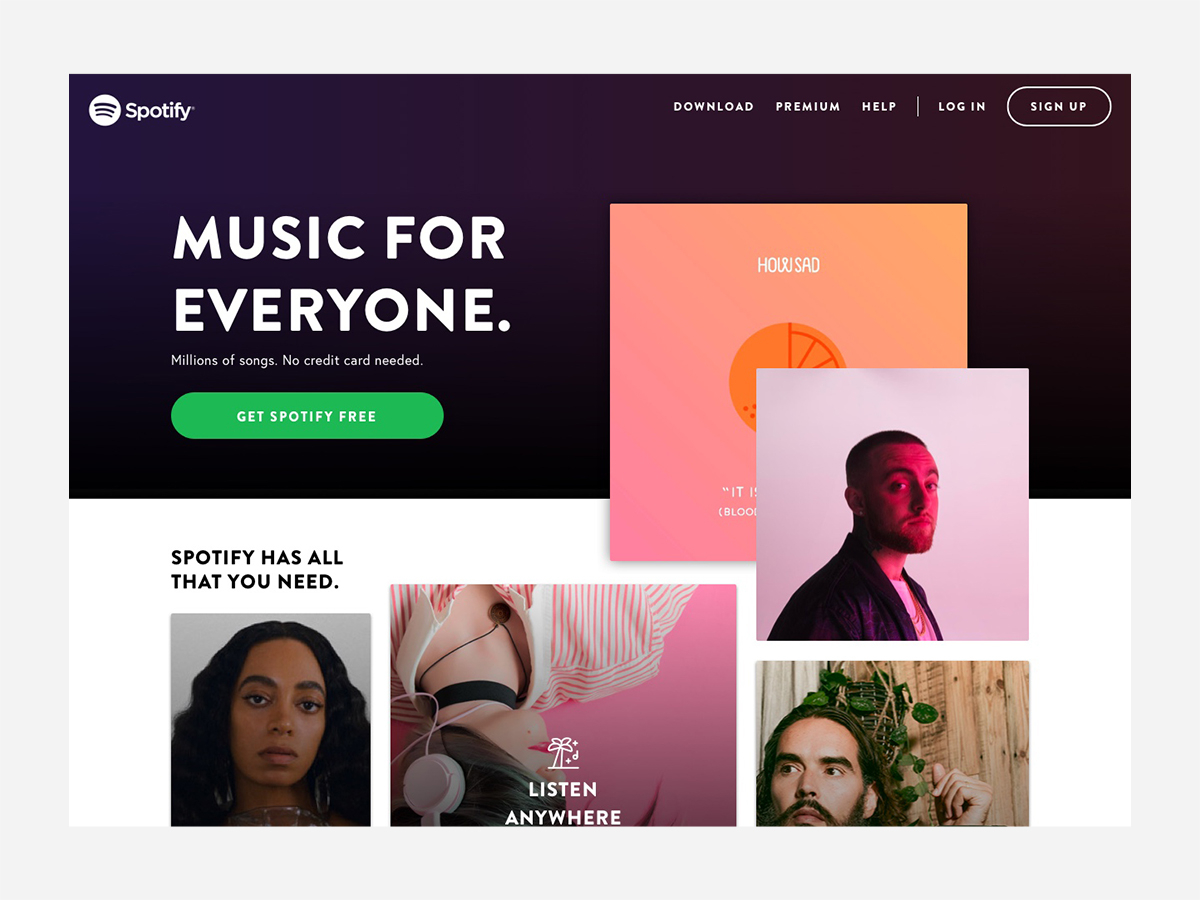This image is a detailed screenshot of the Spotify home page, captured in landscape orientation. The screenshot is framed with a light gray border on all sides. The background of the top section is black, adorned with white text, while the bottom half contrasts as white with black text. There are five overlapping images that span both sections, each showcasing different content.

1. One image prominently features Solange Knowles, suggesting it might be an album cover.
2. Another image appears reminiscent of Russell Brand, although exact identification is uncertain.
3. A third image showcases Mac Miller, seemingly another album cover. He is depicted on top of a peach-colored cover that features an orange drawing and the words "how sad."

The black top section of the page displays the text "MUSIC FOR EVERYONE" in capital letters. Below this heading, there's a prominent green button with white text that reads "GET SPOTIFY FREE." In the upper right corner, menu options are presented in white capital letters, including "DOWNLOAD," "PREMIUM," "HELP," "LOG IN," and "SIGN UP."

Underneath the "MUSIC FOR EVERYONE" line, additional text states, "Millions of songs. No credit card needed," emphasizing the accessibility of Spotify's music library.